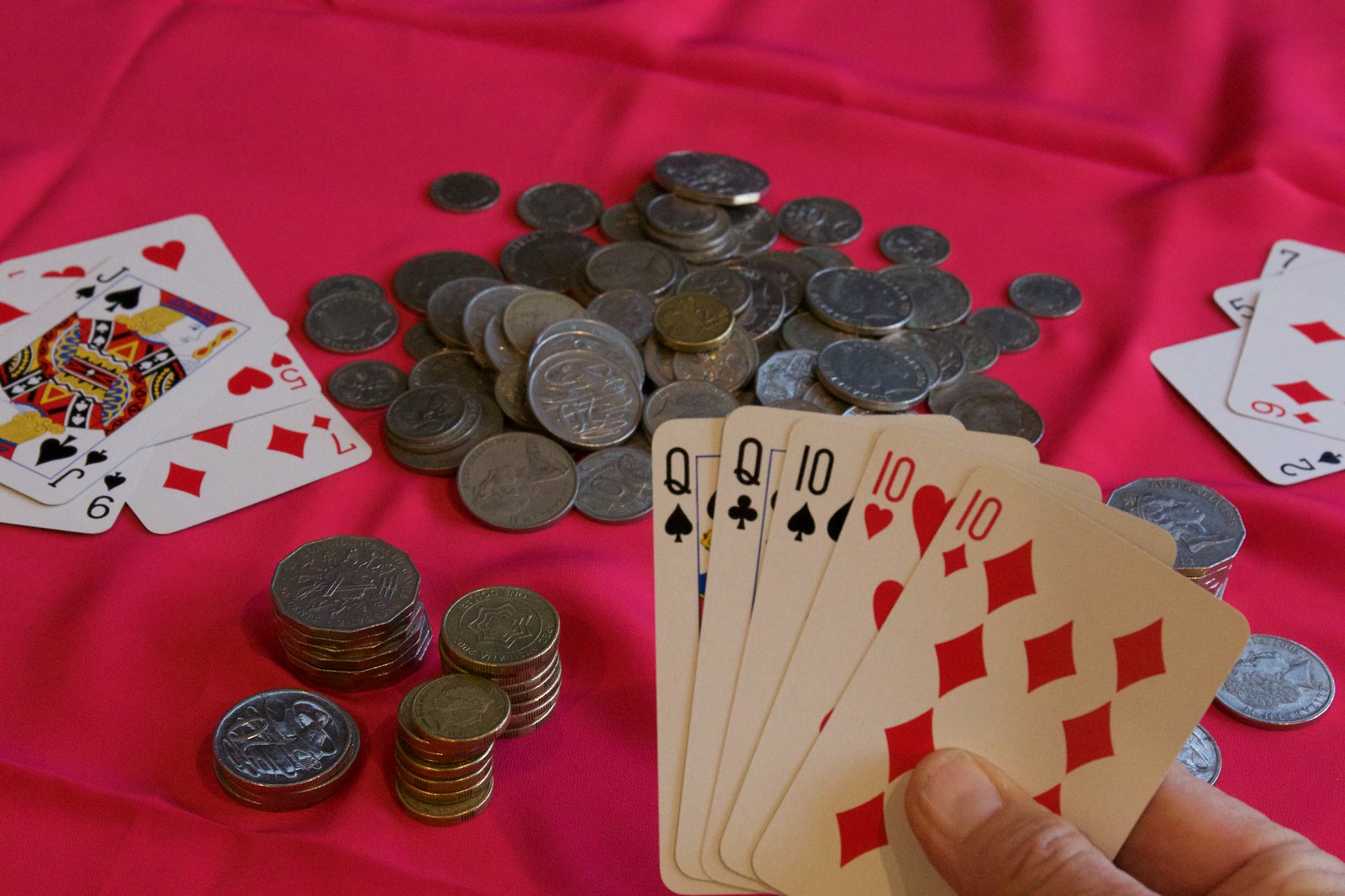This photograph captures an intense moment in a card game, likely poker. Set against a red cloth that presumably covers a table, the scene is centered around a haphazard pile of loose change, interspersed with several neatly organized stacks of coins in the lower left corner. The focal point of the image is a hand of cards prominently displayed, revealing a full house with two queens and three tens, held by a player's thumb and the upper section of their index finger. Surrounding this winning hand are two discarded hands in the upper midsection and right middle of the frame, both appearing to be much weaker in comparison. The strategic arrangement of coins and the compelling card hand suggest a tense but victorious moment in the game, with the player poised to claim a significant win.